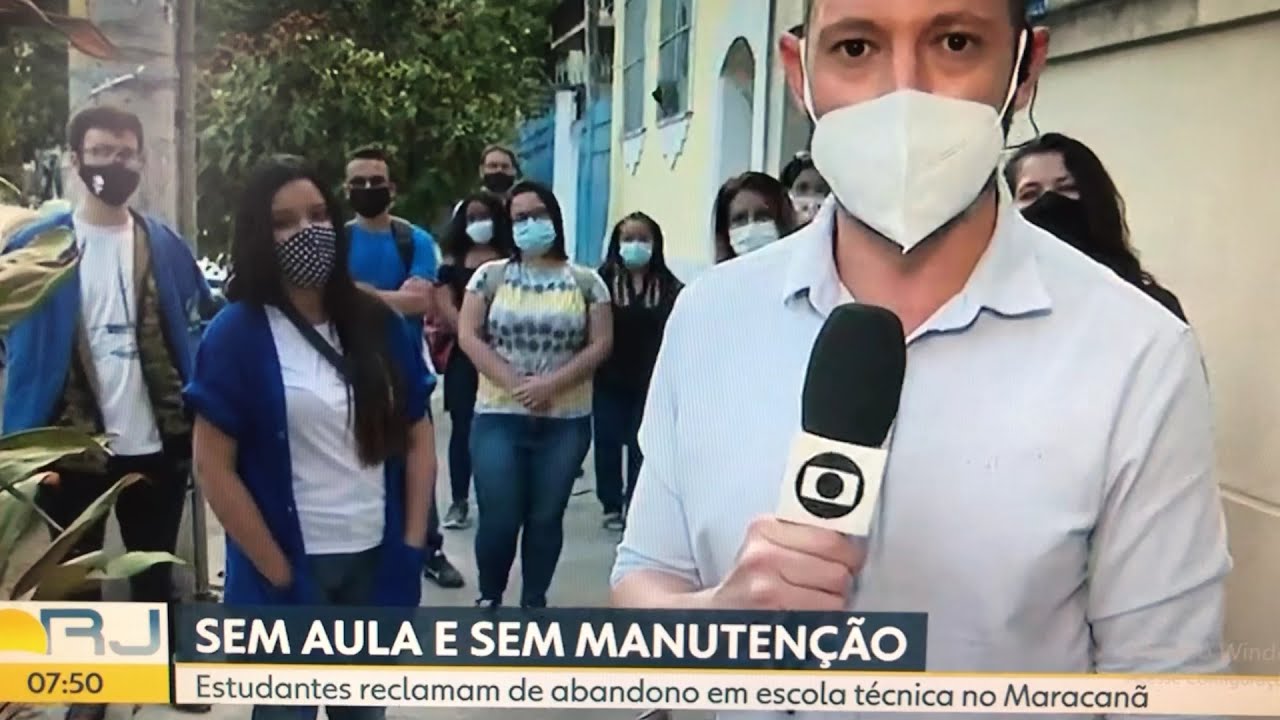The image portrays a journalist standing on the right side of a city sidewalk, wearing a white PPE mask and a light-colored collared shirt, holding a microphone and looking directly at the camera. Behind him, there is a crowd of about ten people, primarily women along with a few men, all wearing masks as well. The setting appears to be outdoors during the day, with a yellowish building on the right and trees in the background. The scene is part of a news broadcast, identifiable by the bottom screen text that includes the logo "RJ" and the time "7.50" in yellow. The remaining text on the banner, likely in Portuguese, indicates this could be a TV screenshot taken during the COVID-19 pandemic. The overall image palette includes colors such as yellow, black, blue, white, light blue, brown, and orange.